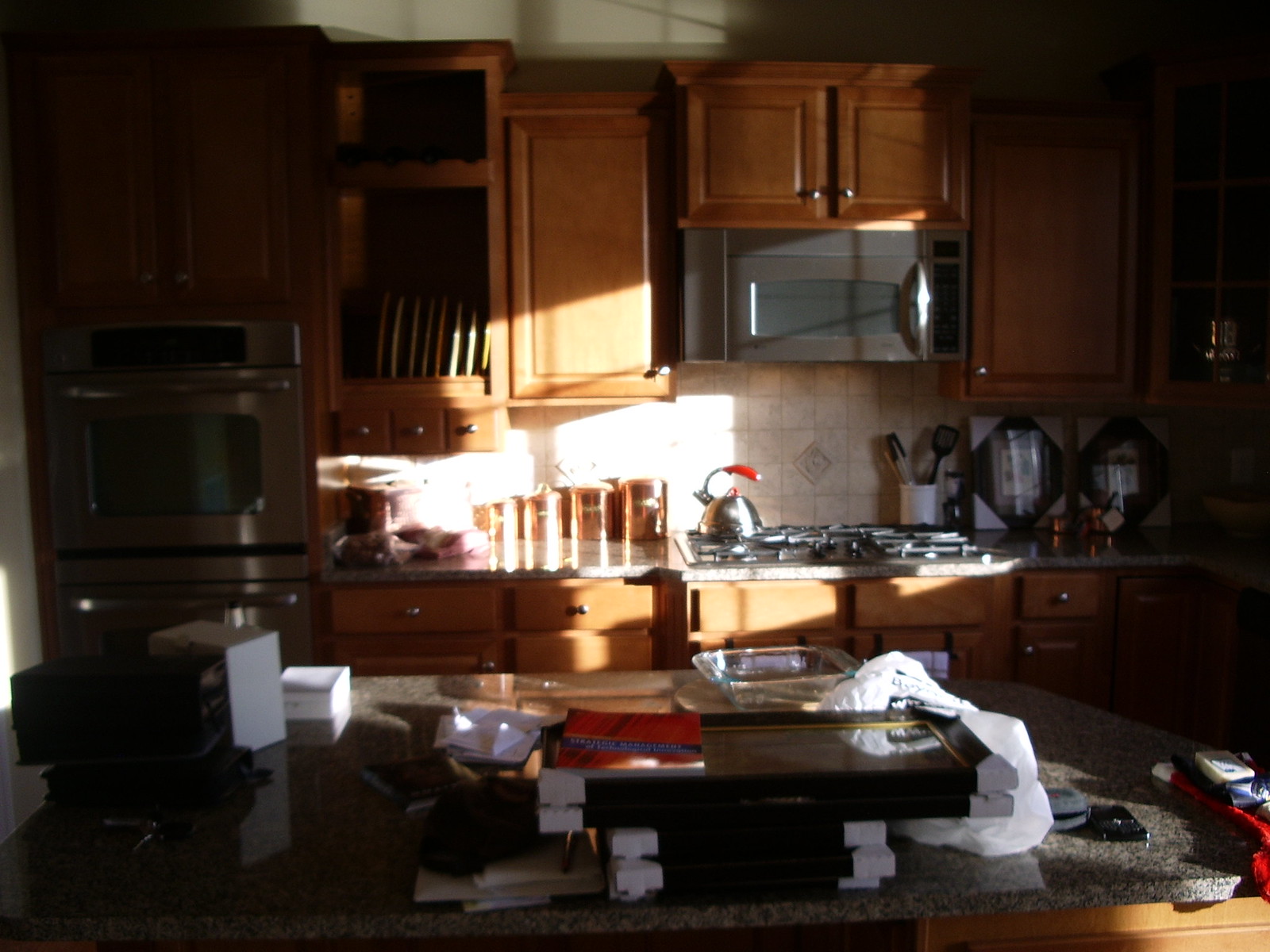The photo captures a chaotic kitchen scene characterized by its cluttered and messy state. In the background, an L-shaped counter is visible, stretching along two walls of the kitchen. This counter is lined with wooden cabinets that add a rustic touch to the space. Prominently featured in this area is a microwave, positioned above a stove range, suggesting a well-used cooking area. Various jars and miscellaneous items clutter the counter surface around the stove, contributing to the overall disarray.

In the foreground, a kitchen island stands independently, providing additional workspace. The entire kitchen is illuminated by a single shaft of light, likely the soft glow of either morning or evening sunlight, which casts a warm, golden hue over the area near the microwave and stove. This light creates a stark contrast, with the brightly-lit spot juxtaposed against the predominantly shadowed and darkened rest of the kitchen, highlighting the lived-in yet neglected state of the space.